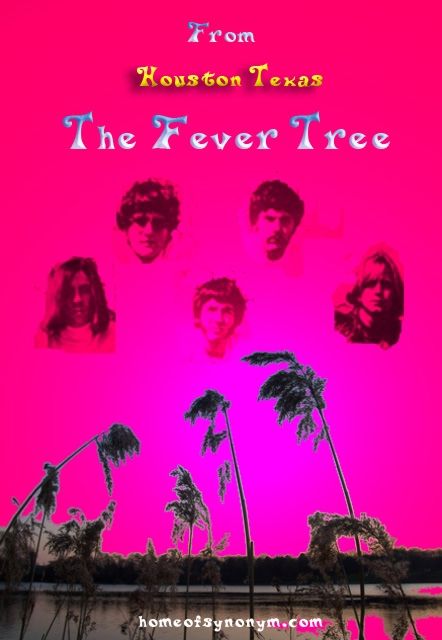This is a vibrant, hot pink computer-animated image designed as a poster or advertisement for the band "The Fever Tree" from Houston, Texas. The top of the image prominently features the phrase "From Houston, Texas, The Fever Tree" in a striking mix of white, blue, and yellow letters. Below this headline, the poster displays five headshots of men, arranged with two at the top and three at the bottom. Each man is white, with varied hairstyles including short dark hair, a mustache, long hair, and blonde hair. The background includes a scenic depiction of lush palm trees, some leaning dramatically, likely suggesting a windy environment, along with green hedges, bushes, and a body of water. At the bottom of the image, the website "homeofsynonym.com" is mentioned, adding a final touch to this detailed and visually engaging promotional material.